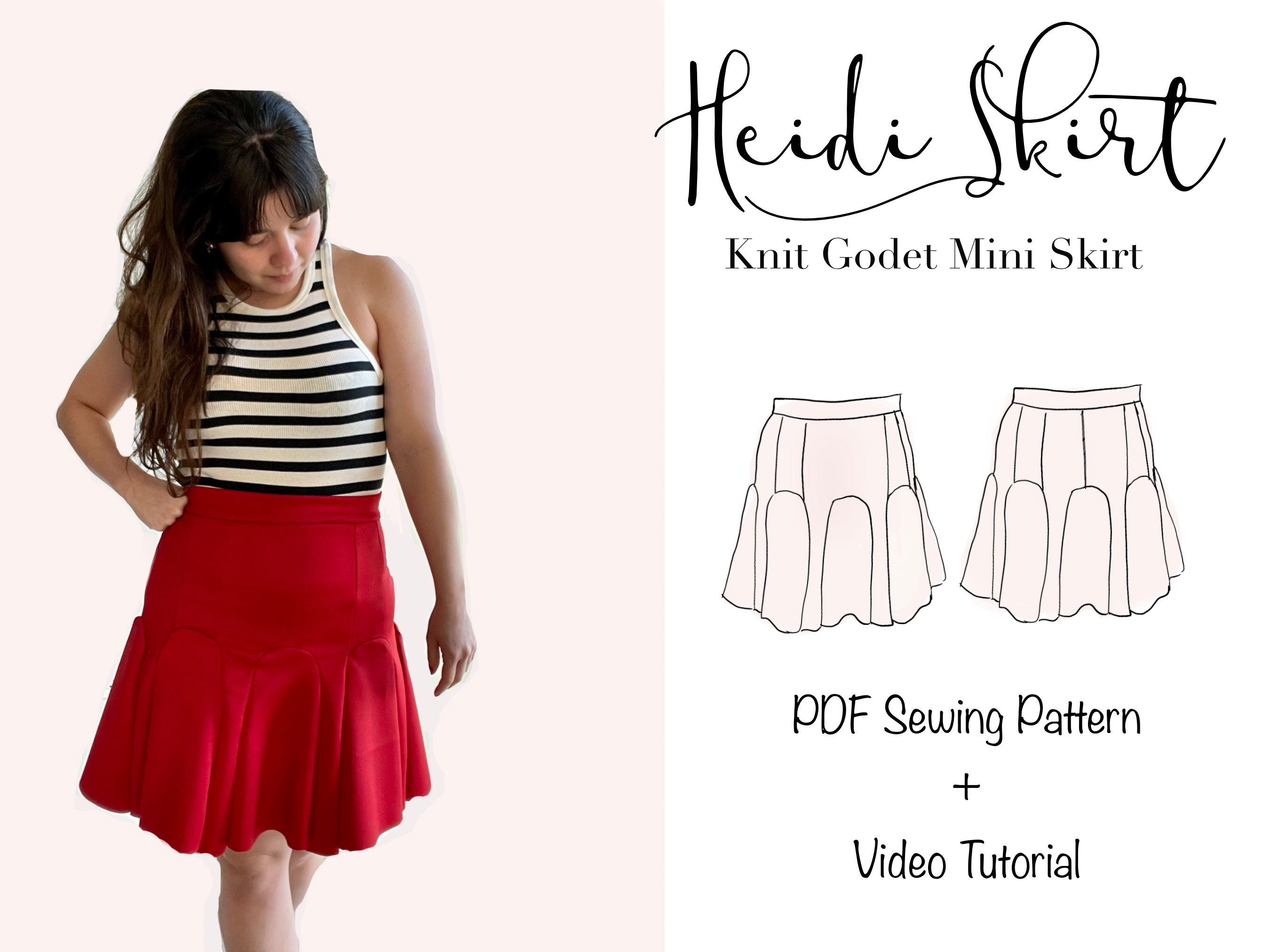The image features a woman with long brunette hair and bangs, styled in a black and white striped tank top or bodysuit and a red skirt. The background is pink. She is looking down towards her midsection and is not making eye contact with the camera. To the right of her, in cursive script, it says "Heidi Skirt, Knit Godet Mini Skirt." Beneath this, there are images of the skirt along with the text "PDF Sewing Pattern plus Video Tutorial." The advertisement presents this specific red skirt as an item for which a PDF sewing pattern and video tutorial are available, illustrating the sewing pattern details and the skirt design.